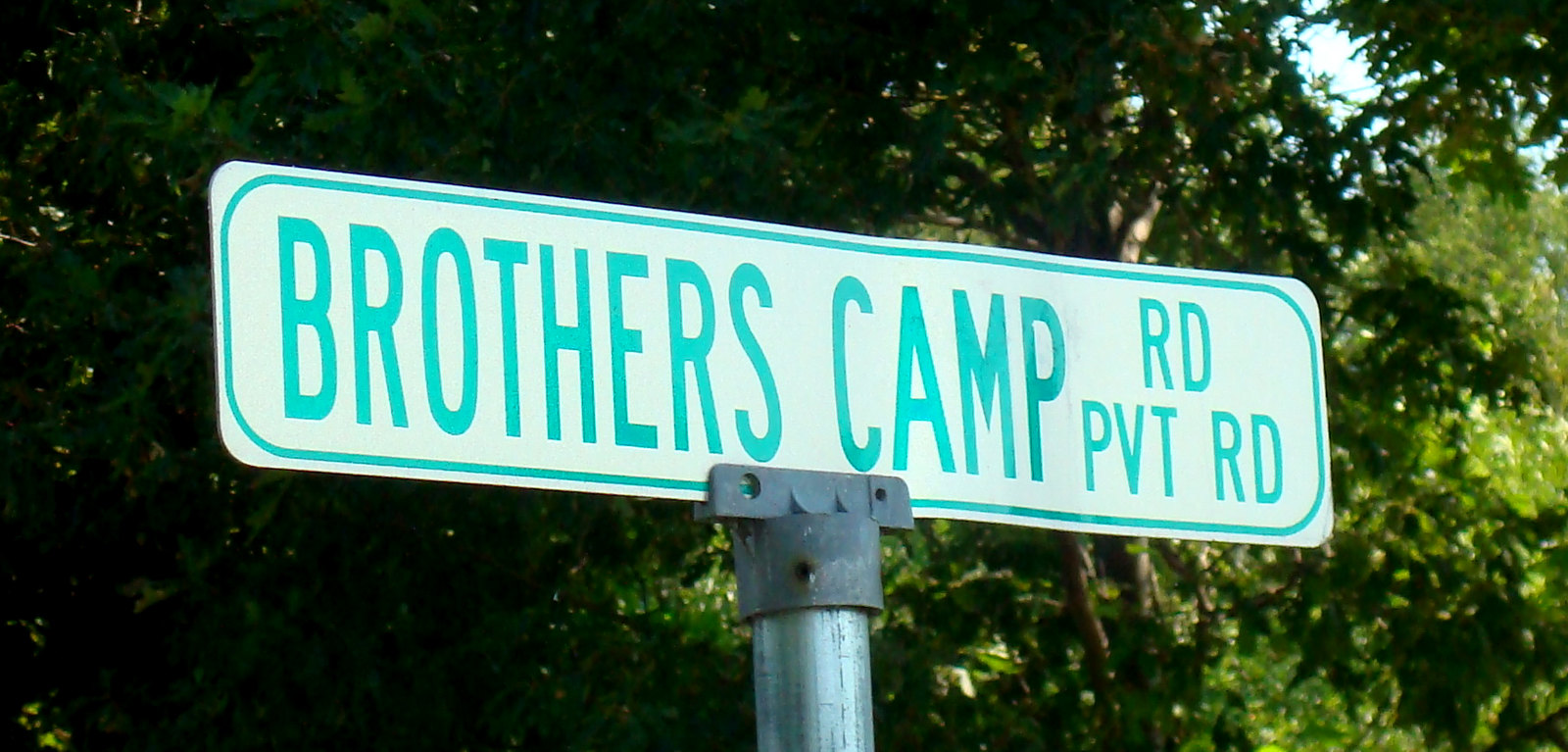This photograph captures an upward view of a street sign set against a backdrop of densely packed, mature trees with exuberant green foliage. A small patch of blue sky peeks through the verdant canopy, adding a splash of color to the scene. The street sign is mounted on a sturdy, silver metal pole that extends vertically from the ground. Attached to the top of the pole is a bracket that securely holds a long, rectangular white sign with slightly rounded corners. The sign displays the text "Brothers Camp Road, Private Road" in an appealing aqua, bluish-green font, clearly indicating the name of the road and its private status. The interplay of natural and human elements in this image creates a harmonious visual composition.